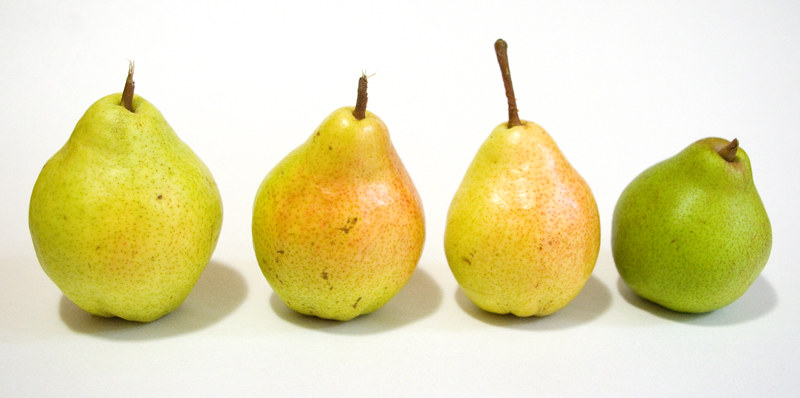This is a detailed photograph capturing a sequence of four plump and rotund pears, each in varying stages of ripeness. They are neatly arranged on a white surface with a slightly off-white bottom, against a clean white background. Starting from the left, the first pear is the largest and stands straight up. It is a light green with small brown specks and has a stem that appears uneven, as though it has been broken off. To its right, the second pear is slightly smaller, leaning to the right, and showcases a yellow-green hue with orange and brown freckles. Its stem is the longest among the four. The third pear is more yellow with orange tones, exhibits brown specks, and stands almost straight up with its stem leaning slightly to the left. The smallest pear on the far right is the darkest green, featuring a few brown spots and leans to its right with a very short, tiny brown stem. Each pear's distinct color and position create a visual journey from left to right, reflecting their diverse stages of ripeness.